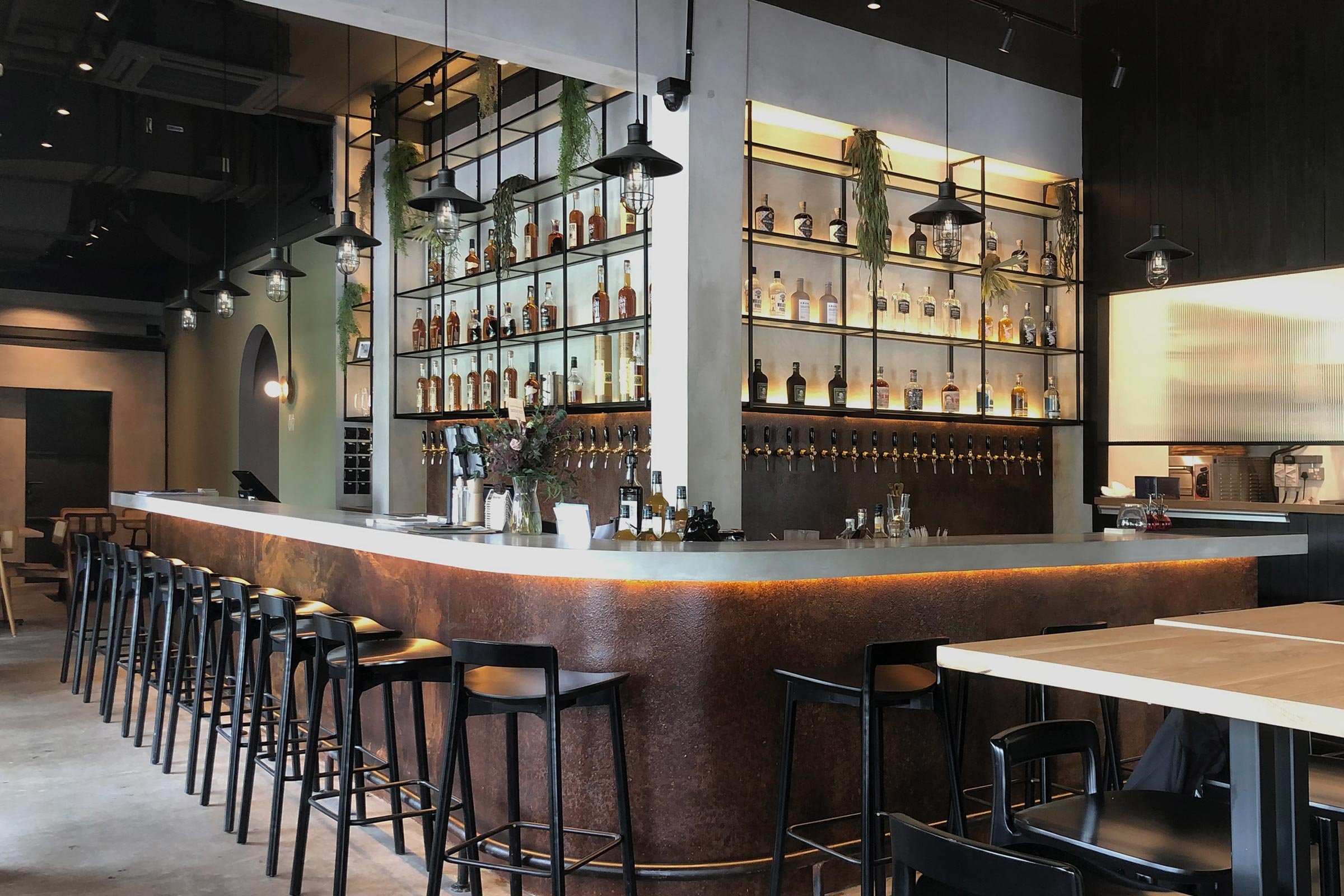The image depicts an upscale, meticulously clean bar radiating a refined Mediterranean or Spanish vibe. The bar, possibly at opening or closing time given its pristine condition and absence of patrons, is bathed in natural light, suggesting early day hours. The bar's design is modern and sophisticated, featuring a sleek, marble countertop with a light running underneath, paired with a wooden base. 

Rows of uniform and evenly spaced spirits line the shelves behind the bar, accompanied by an impressive array of beer taps, perhaps around twenty or more on either side, indicating a vast selection. The bar's seating comprises low-hanging, metal black stools without backrests, providing minimal support. These stools are also found around bar-height tables in the foreground.

Decorative elements include clear glass cases showcasing various liquors and industrial-looking overhead lights, which likely contribute to a dim, ambient setting in the evening. The overall atmosphere is one of calm anticipation, as if the space is ready to welcome guests at any moment.